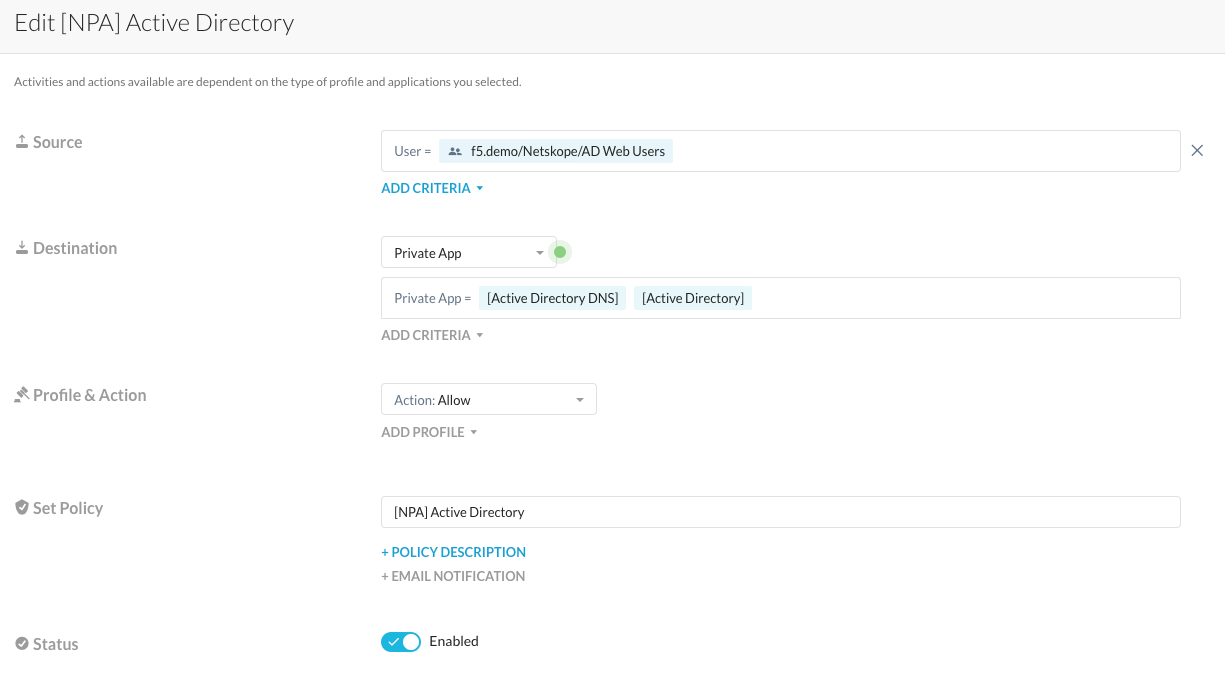In this image, the interface for editing an NPA (Network Protection Application) Active Directory policy is displayed. At the top, the title reads "Edit [NPA] Active Directory," indicating the policy type being configured. The policy's available activities and actions are contingent on the selected profile and applications.

The image is divided into three main sections: Source, Destination, and Profile & Action.

1. **Source Section**:
   - There is a search box with the entry "user = F5.demo/Netscope/AD web users".
   - Below the search box is an "Add Criteria" dropdown menu for further refining the source criteria.

2. **Destination Section**:
   - This section features a dropdown menu where "Private App" is selected.
   - A box beneath this dropdown shows the condition "private app = [Active Directory DNS] [Active Directory]".
   - Like the Source section, there is an "Add Criteria" dropdown menu provided for additional specifications.

3. **Profile & Action Section**:
   - This section includes a dropdown labeled "Action: Allow," indicating that the action for this policy is to allow access.
   - There is also an "Add Profile" dropdown for associating a profile with the action.
   
At the bottom of the interface, there is a "Set Policy" statement reading "[NPA] Active Directory". Additionally, there is an area for policy description and email notifications, presumably for administrative use or alerts.

Finally, the "Status" section features a toggle that has been set to "Enable," activating the policy.

This comprehensive interface allows for detailed management and customization of access policies within an Active Directory environment.